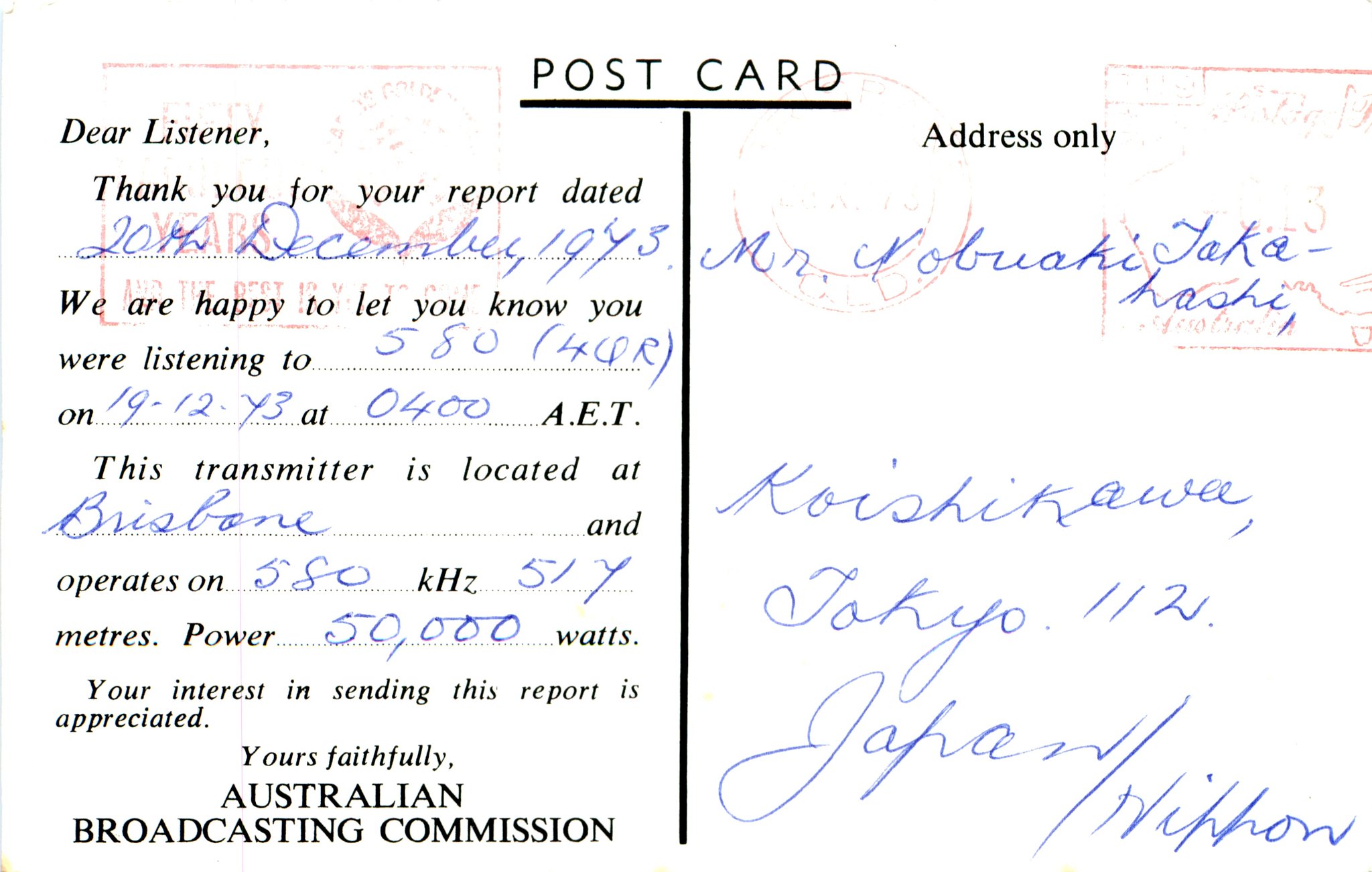A vintage postcard features a faded red stamp ink marking and the word "Postcard" prominently printed at the top center, accompanied by a horizontal black line underneath and a vertical black line bisecting the card into two halves. On the left side, a printed message reads: "Dear Listener, thank you for your report dated," followed by the handwritten date "20th December 1943" in blue ink. The message continues, expressing gratitude and confirming the listener was tuned into "584QR" on "19-12-43 at 0400 AET," with details about the transmitter location and specifications: "This transmitter is located at Brisbane and operates on 580 kilohertz, 517 meters, power 50,000 watts." It signs off with "Your interest in sending this report is appreciated. Yours faithfully, the Australian Broadcasting Commission." Meanwhile, the right side is designated for the recipient’s address, written in blue ink as "Mr. Kobukari Jake Hashi," followed by "Korehashikawa, Tokyo 11 to Japan / Hilton."